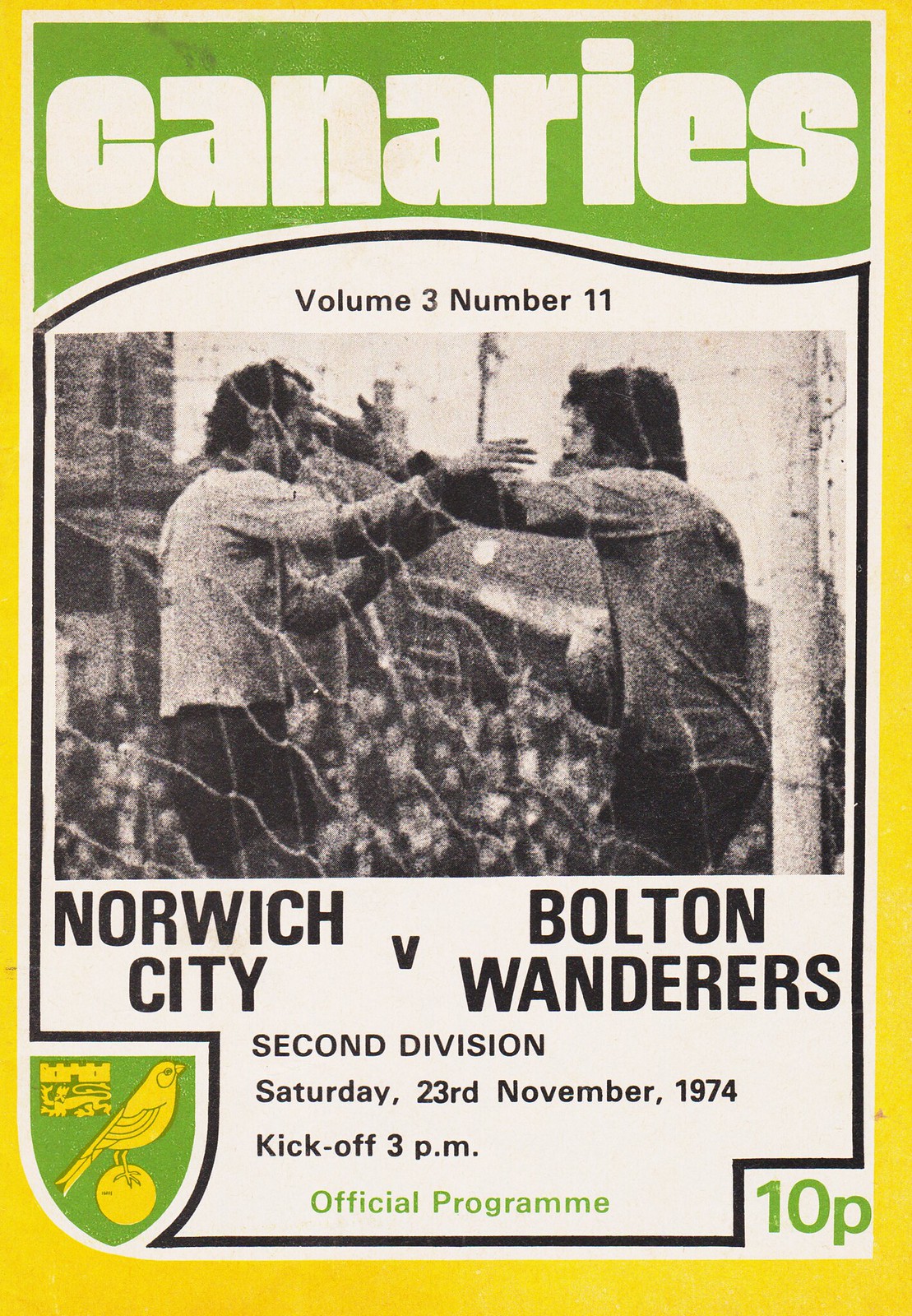This detailed caption synthesizes the shared and repeated details from all three sources:

This vivid yellow page from a 1974 soccer club program features a wavy green banner at the top with "Canaries" prominently displayed in white. The focus of the page is an inset black and white photograph of two smiling soccer players, apparently mid-embrace, standing in front of a net. Labeled "Volume 3, Number 11," the program is titled "Norwich City vs. Bolton Wanderers, 2nd Division," and specifies the match took place on Saturday, 23rd November 1974, with a kickoff at 3pm. "Official Program" and the price, "10p," are also included. In the lower left-hand corner, a shield-shaped logo features a bird perched on a soccer ball beside a crest of a lion, suggesting this is all official memorabilia from the game.